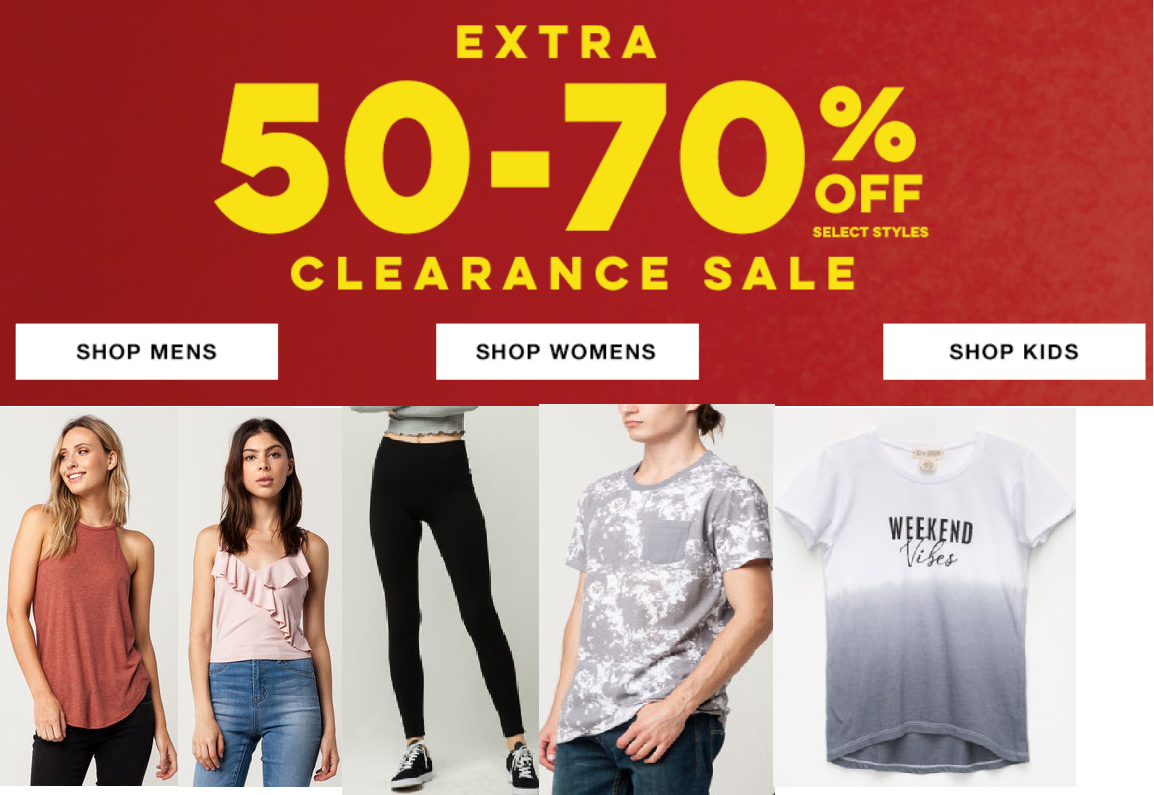The image is a sale notification featuring a vibrant red background with bold, yellow text prominently announcing a "50% to 70% OFF" discount. Above this prominent message, the word "EXTRA" stands out, and below it, the phrase "CLEARANCE SALE" is displayed. To the right of the percentage discount, it is noted that the offer applies to "select styles."

The lower section of the image contains clickable white buttons with black text, directing shoppers to different sections: "Shop Men's" on the left, "Shop Women's" in the center, and "Shop Kids" on the right.

Beneath these buttons, there are photos of various models showcasing the sale items:
1. Two women both wearing sleeveless tops; one in a burnt orange shirt paired with black pants, and the other in a pink shirt with blue jeans. Both women have visibly tan skin tones, one with blonde hair and the other with brown hair.
2. A close-up shot of another model from the waist down, wearing black leggings similar to yoga pants, paired with black and white tennis shoes.
3. A partial view showing only the head up to the nose of a person dressed in a gray and white splotchy short-sleeved t-shirt and blue jeans.
4. A t-shirt displayed on its own, white on top and gray on the bottom, with the phrase "Weekend Vibes" printed on it in short-sleeved style.

Noticeably detailed and vibrant, the image is designed to attract attention and promote the sale despite the absence of store-specific information.